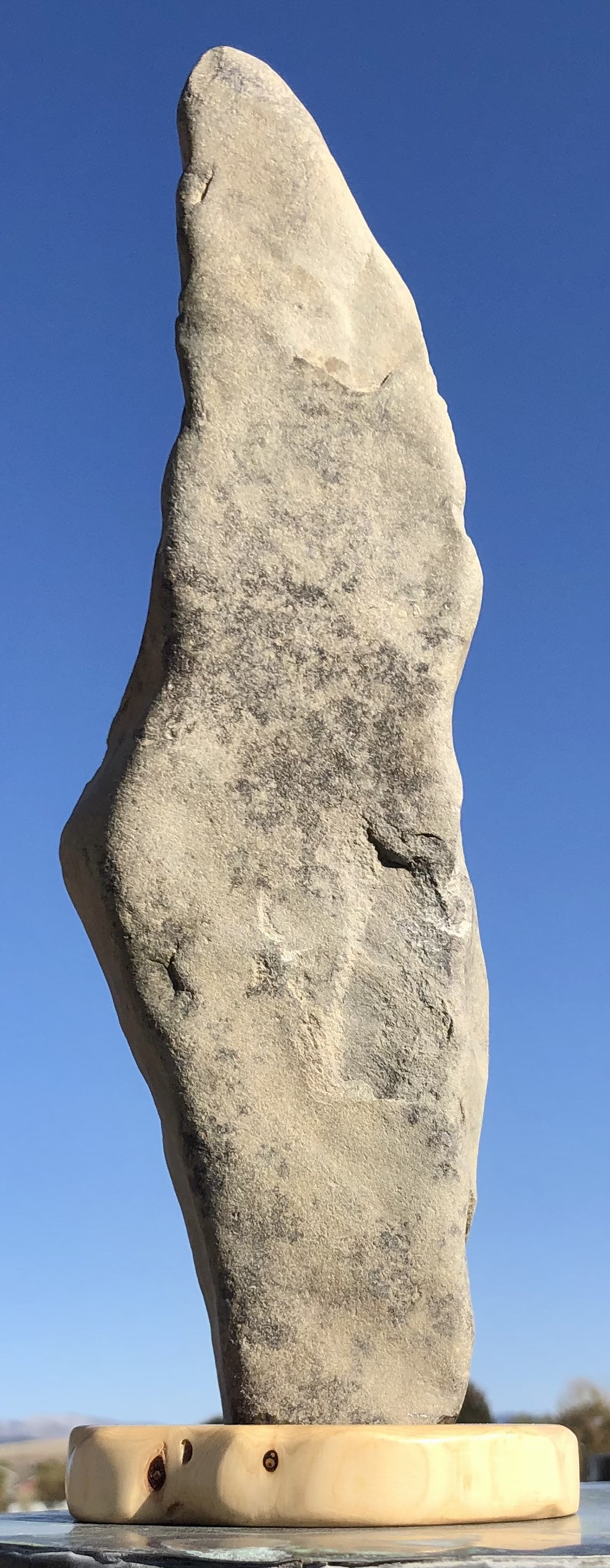The photograph features a vertical, tall rock resembling a sculpture or art piece, prominently extending skyward against a backdrop of a clear blue sky. The rock, lacking distinguishable carvings, is predominantly gray and tapers into a shape that recalls both a spearhead and a scythe. It sits on a distinctive off-white base, which is textured with dent-like features reminiscent of bone. The entire setup suggests the rock is mounted on a platform or table. In the blurred background, there are vague outlines of trees or hills, emphasizing the outdoor setting and the rock's imposing, statue-like presence.